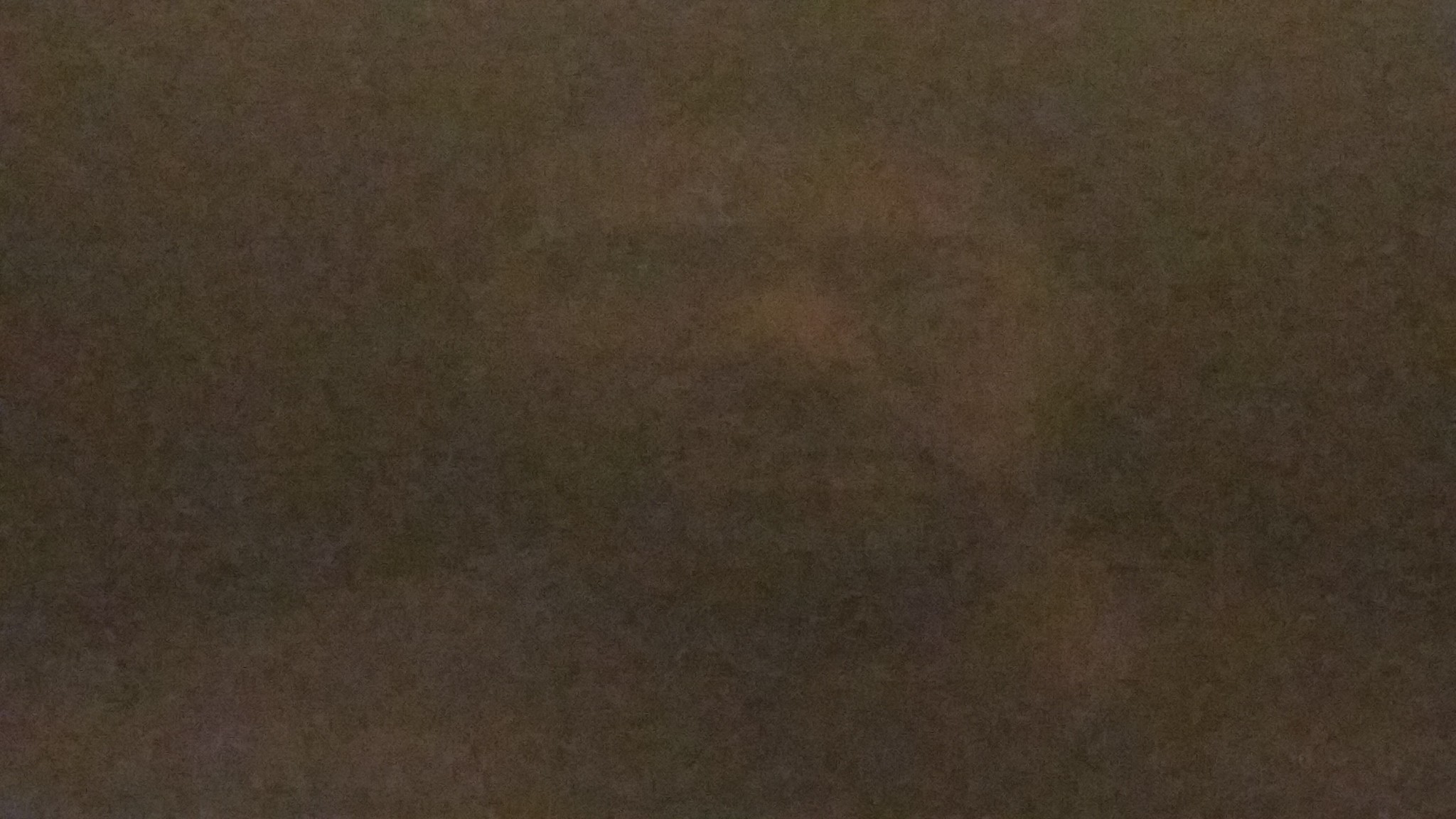The image is a blurry, grainy, and spooky photo featuring a faint outline of a man's face and shoulders. Predominantly dark, with shades of black and dark brown, the man's figure blends almost imperceptibly into the background. At first glance, the picture might appear as a mere black square, but upon closer inspection, you can discern the central figure—a man positioned directly in the middle, looking straight forward. His dark, short hair is somewhat noticeable, as are the vague shapes of his eyes, nose, and mouth, though they are not well-defined due to the noise and blur. His shoulder line is faintly visible from the left bottom to the right bottom of the image, and what may be his neckline is similarly blended into the background. The blurry and out-of-focus nature of the photo, combined with the low contrast, gives the impression that the man's face stretches unnaturally, adding to the eerie vibe.